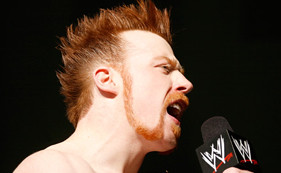The image depicts a detailed and vivid portrait of WWE wrestler Sheamus, captured mid-speech, with his mouth open as he speaks into a handheld microphone. The focus of the photo is exclusively on the head and top shoulders of Sheamus, a white male in his 30s or 40s. His bright ginger hair is styled into a distinctive mohawk, and his facial hair includes a thin beard with shaven cheeks, complemented by a mustache and a small soul patch. Not wearing a shirt, he is depicted in a profile view, emphasizing the right side of his face. The black microphone in his hand prominently features the WWE logo, a white "W" with a red line underneath it, positioned on its square base. The photo is taken against a pitch-black background, likely in a studio, emphasizing the wrestler's animated expression and distinctive appearance. The image is in full color and sharply illuminated, providing a clear and dramatic depiction of Sheamus in action.